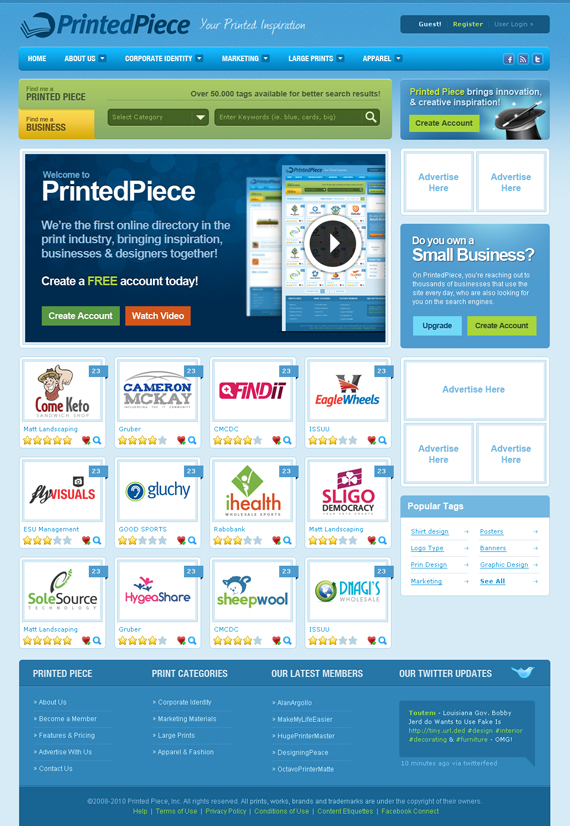The image showcases a promotional webpage designed with a visually appealing blend of blue hues and a splash of olive green. On the left side of the header, the bold title "Printed Piece" stands out prominently in a large font, featuring two shades of blue with the word "Printed" appearing lighter than "Piece." Directly beneath it, the phrase "Your Printed Inspiration" is elegantly scripted in cursive white text.

On the right side of the header is a vertical bar containing navigation options: "Guest," "Register," and "User Login," each paired with a right-facing arrow. The "Register" option is highlighted in yellow, while "Guest" is in white and "User Login" is in a blue similar to the background, blending into the button area.

Above this section, a light blue background spans across the top of the webpage, where a series of navigation options are listed horizontally, each accompanied by a drop-down menu. These options include: "Home," "About Us," "Corporate Identity," "Marketing," "Large Prints," and "Apparel." On the far right of this blue bar, there are icons linked to social media platforms, including Facebook, though the identities of the other two icons are unclear.

Below the header, there's a horizontally oriented, light olive green rectangle that runs longer than it is tall. Positioned in the upper left corner of this rectangle is the phrase "Find me a Printed Piece." The remainder of the page continues with the light olive green theme. It is emphasized that there are over 50,000 tags available for refining search results.

Within this olive green section, there is a darker olive green button labeled "Select Category" with an adjacent drop-down menu. To the right of this button, there is a search field with placeholder text suggesting keywords like "blue," "cards," and "big," complemented by a magnifying glass icon indicating the search function.